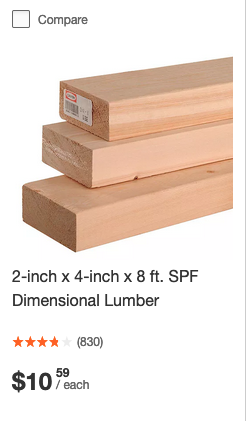A screenshot detail from an e-commerce website, such as Lowe's or Home Depot, showcases a product listing for 2x4 SPF dimensional lumber. The image, oriented vertically, features a white background with the primary focus on a stack of three 2x4 boards arranged in a stepped formation. The top board is the furthest back, the middle board slightly forward, and the bottom board extending the furthest, creating a staircase effect. A plastic label is stapled to the end of the top board, while the others remain unlabeled.

In the upper left corner of the image, there is a checkbox labeled "Compare," allowing users to compare this product with others, though it remains unchecked. Beneath the image, the product is described as "2-inch x 4-inch x 8-foot SPF dimensional lumber," with hyphens appropriately placed between numeric values and measurement units.

Below the description is a star rating indicator, showing just under four yellow stars out of five, based on 830 customer ratings. The price is prominently displayed in bold black numbers: $10.59, with the dollar sign significantly larger and the '59' raised slightly like a superscript. The price is followed by the phrase "per each."